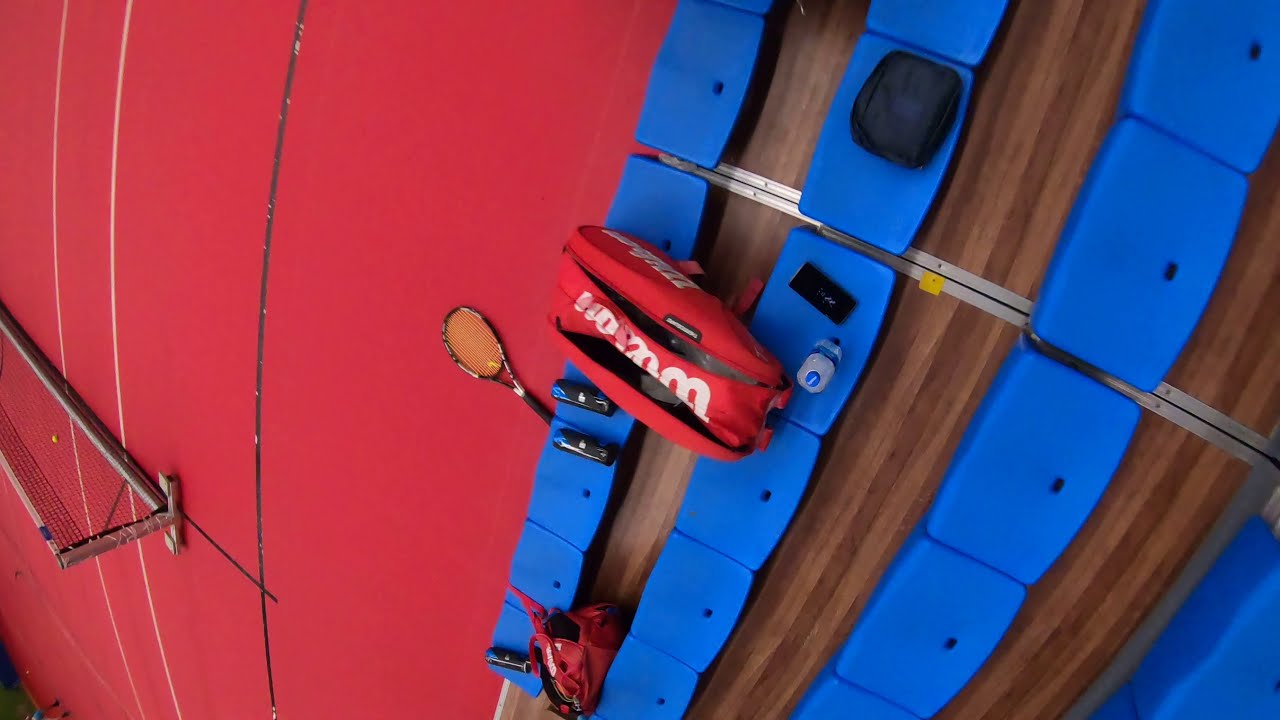The image is a top-down view of a tennis court with a red surface featuring white lines, and a portion of the tennis net visible in the lower left corner. Centrally positioned on the court are blue bleacher seats resting on a wooden platform, and these bleachers appear to be partially folded. Atop the front row of these seats sits a red gym bag with indecipherable writing, partially obscured by a black strap and a zipper. Stretching from the center towards the left is a black-handled tennis racquet with orange strings. Adjacent to the racquet and close to the bleachers lie two small black cylindrical objects with blue tips. The photo composition suggests it might be rotated sideways.